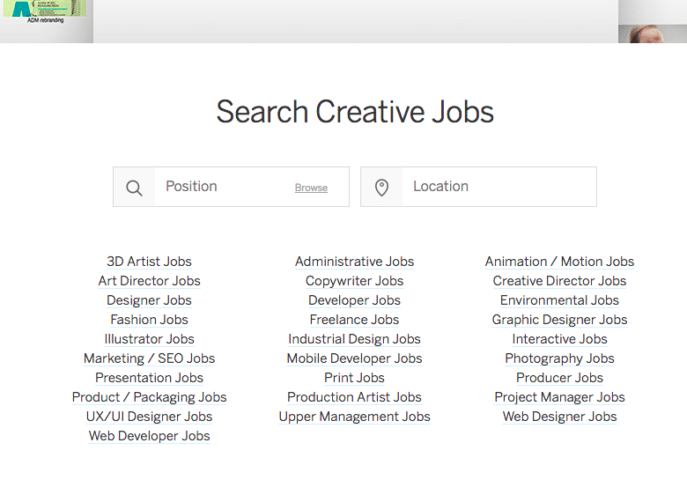The image features a streamlined user interface for a creative job search platform. At the top of the screen, a long gray bar stretches horizontally. On the left side of the bar, there is a green square. Towards the right side of the bar, there is a glimpse of someone's forehead sporting blondish-brown hair. Below this bar, the words "Search Creative Jobs" are prominently displayed in bold black text. Adjacent to the text, on the left, is a rectangular search box containing a magnifying glass icon, and beside it, the word "Browse" is underlined.

Further down, another section showcases a search filter with a circular icon that narrows to a point, indicative of a location pin. Next to this icon, the word "Location" appears.

The job categories are organized into three neatly aligned columns. The first column lists: 
- 3D Artist Jobs
- Art Director Jobs
- Designer Jobs
- Fashion Jobs
- Illustrator Jobs
- Marketing Jobs
- Web Developer Jobs

The second column includes:
- Administrative Jobs
- Copywriter Jobs
- Developer Jobs
- Freelance Jobs
- Industrial Design Jobs
- Mobile Developer Jobs

The third column features:
- Animation/Motion Jobs
- Creative Director Jobs
- Environmental Graphic Designer Jobs
- Interactive Jobs
- Photography Jobs
- Producer Jobs
- Project Manager Jobs
- Web Designer Jobs

Each job category is a clickable link, offering users an extensive variety of positions within the creative industry.